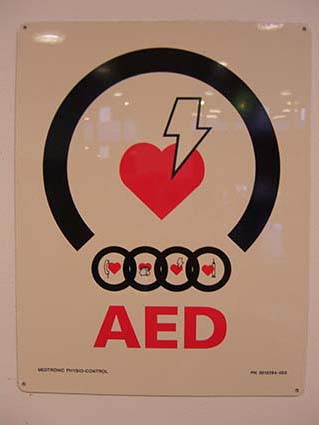This image features a glossy, shiny sign attached to a wall. Dominating the sign is a near-complete black circle at the top, with a segment missing at the bottom. Centered within this circle is a vivid red heart intersected by a lightning bolt on its right side. Below the incomplete section of the black circle, four smaller interconnected circles, each containing heart images, are prominently displayed. Underneath these elements, in bold red capital letters, the abbreviation "AED" is clearly visible, signifying the presence of an Automated External Defibrillator, a critical device for managing cardiac arrest emergencies. Reflections of light on the glossy surface of the sign add a visual depth to the image.